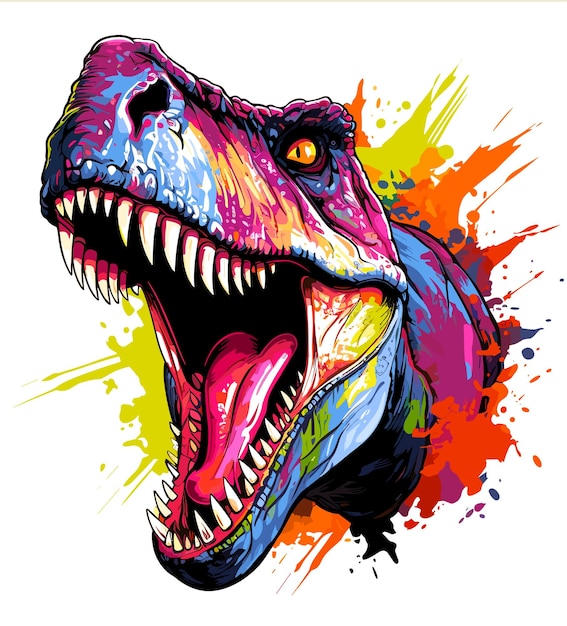This vibrant and striking illustration depicts a Tyrannosaurus rex head bursting through the page with an explosion of color. The T-Rex is depicted in a dynamic, aggressive stance with its mouth wide open, revealing rows of white teeth that appear to be streaked with red at the tips, giving the impression of blood. Its pink tongue is prominently visible amidst the open maw. The left eye of the T-Rex glares out, painted in a vivid orange color, and its nostrils are also distinctly colored.

The T-Rex is rendered in a dazzling array of day-glo colors, reminiscent of a tie-dye pattern, with hues of red, yellow, orange, turquoise, maroon, magenta, neon blue, lime green, and bright orange blending seamlessly across its form. The upper part of its snout through to the top of its head is primarily turquoise and orange, while the bottom half of its body showcases deep blues. A maroon splotch further accents its textured skin.

Behind the T-Rex, a chaotic and colorful paint splotch background enhances the sense of depth and motion, making it look as though the dinosaur is bursting through the canvas towards the viewer. This stylistic backdrop adds a layered effect, making the artwork appear almost three-dimensional and lending it a blend of photorealism with artistic flair.